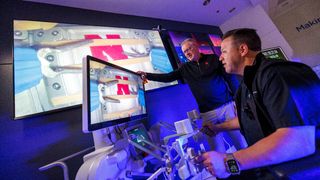This is a small, horizontal color image depicting a dimly lit control room with two men deeply engaged in operating equipment. Both men, dressed uniformly in black shirts, are focused on a smaller monitor placed on a cluttered desk. The monitor displays the same graphics projected on a much larger screen mounted on the wall behind them. The graphics include a large red "N" and a robotic device, possibly controlled by the equipment in the room. One man, seated at the desk, manipulates some controls while the other points at the screen, attentively observing the actions. The room, illuminated by a purple cast of light, suggests a serious atmosphere, possibly a lab or a control station for a mechanized device or TV show. Despite the darkness, their concentrated expressions and synchronized actions hint at the technical precision of their tasks.